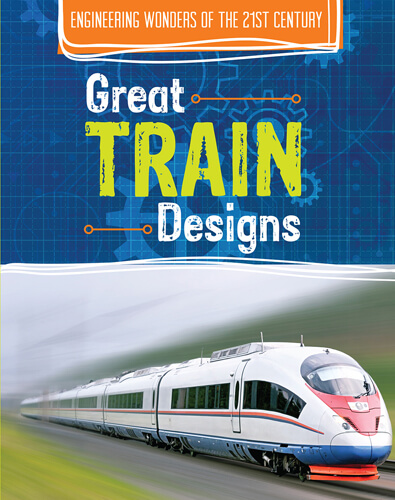This is an image of a digitally created cover, possibly for a book or a magazine, titled "Engineering Wonders of the 21st Century: Great Train Designs." The cover is divided into two halves. The upper half features a blueprint-style background in blue, adorned with interlocking gears and sprockets. The title "Great Train Designs" is prominently displayed in white and green print, while the phrase "Engineering Wonders of the 21st Century" is enclosed in an orange box at the very top. The bottom half of the cover showcases a futuristic bullet train, painted white with a streamlined, tapered nose and a red and blue stripe running down its length. The train, which appears to be electric, is depicted with about five or six passenger cars and is shown moving at high speed on a rail track under a gray sky. The number "614" is visible on the nose of the train, enhancing the sense of specificity and detail. The overall presentation emphasizes the combination of elegant design and modern engineering.